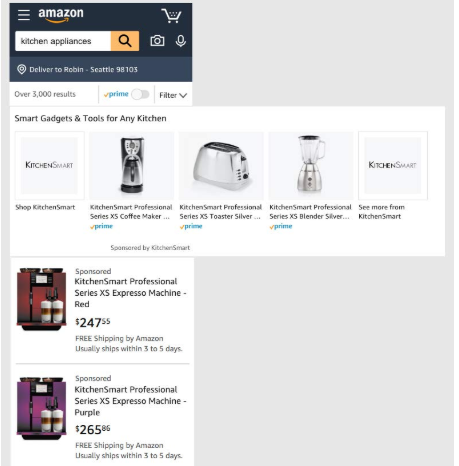The image is a vertical rectangle featuring a screen grab from Amazon's website. The entire frame has a light gray background. The left half of the frame prominently displays the Amazon logo, a search bar, and various product listings. Just above the center of the frame, a product window extends to the right side, showcasing items laid out horizontally next to each other. This window is flanked by the light gray background above and below it on the right side. Below this central window, two additional product listings are displayed: the Kitchen Smart Professional Series XS Espresso Machine, available in two colors—red and purple. The red espresso machine is priced at $247.55, while the purple one costs $265.86.